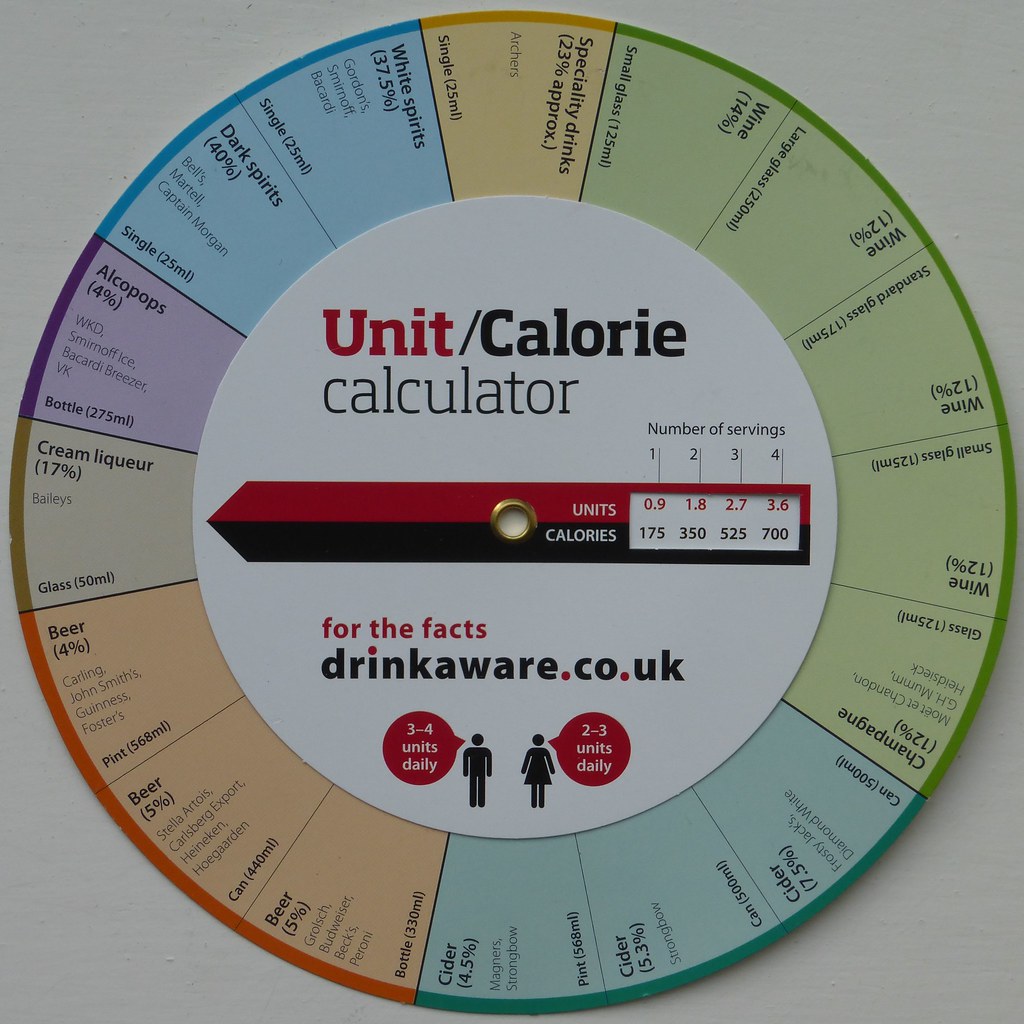The photograph features a detailed dial designed as a Unit/Calorie Calculator. The center of the dial displays a white circle with the text "unit" in red and "calorie" in black, underneath which it reads "calculator." Surrounding this central circle, there's a scale marked with the numbers one to four, labeled as "number of servings." A red and green arrow points to the left, just above text that reads "for the facts" in red font, and below that, "drinkaware.co.uk" in black.

Adjacent to this, black silhouettes of a man and woman provide daily recommended alcohol unit guidelines: three to four units for men and two to three units for women. Encircling the dial are various types of alcoholic beverages, color-coded and ranging from wines and ciders to beers, cream liqueurs, and spirits, each labeled with corresponding alcohol percentages, which span from 4% beer to 40% spirits. The dial functions by turning to align with specific drinks, revealing how many units and calories are in up to four servings through a small window.